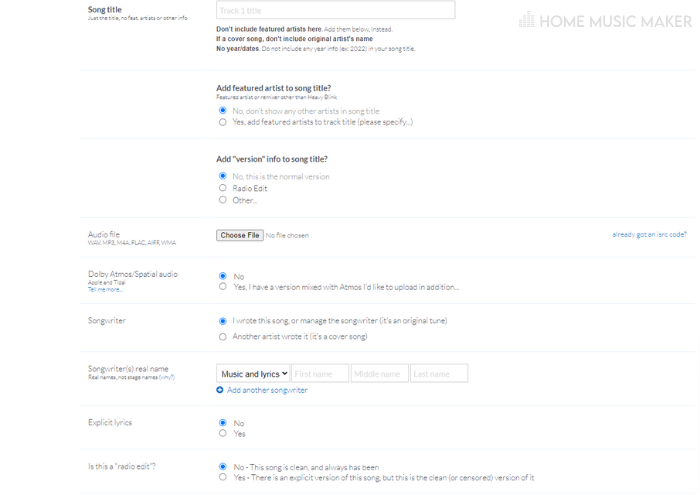The image depicts a user interface, likely the settings area for an application or website related to music creation. The background is solid white, giving a clean, uncluttered aesthetic without visible edges. The layout is slightly wider than it is tall, but the difference in dimensions is minimal.

In the upper left corner, there's a prominent title labeled "Song Title" in large text. Directly below this title is a line of text that's difficult to decipher. Adjacent to it on the right is an empty input box with placeholder text that reads "Track One Title," indicating where users can type in information.

The upper right corner features four vertical bars resembling a bar graph, rendered in light gray. To their right, in all caps, is the text "HOME MUSIC MAKER." 

Below this section, there's a small block of three lines of text, which presents some instructions and guidelines, although parts of it are difficult to read. The first line clearly says "Don't include featured artists here," followed by smaller, less legible text. The second line advises "If a cover song, don't include the original artist's name." The final line notes "No year/dates," with some additional unreadable text following.

A horizontal light blue bar demarcates the end of this first section. Beneath it, another section appears, titled "Add featured artists to song title?" with options to select "Yes" or "No" via checkboxes below.